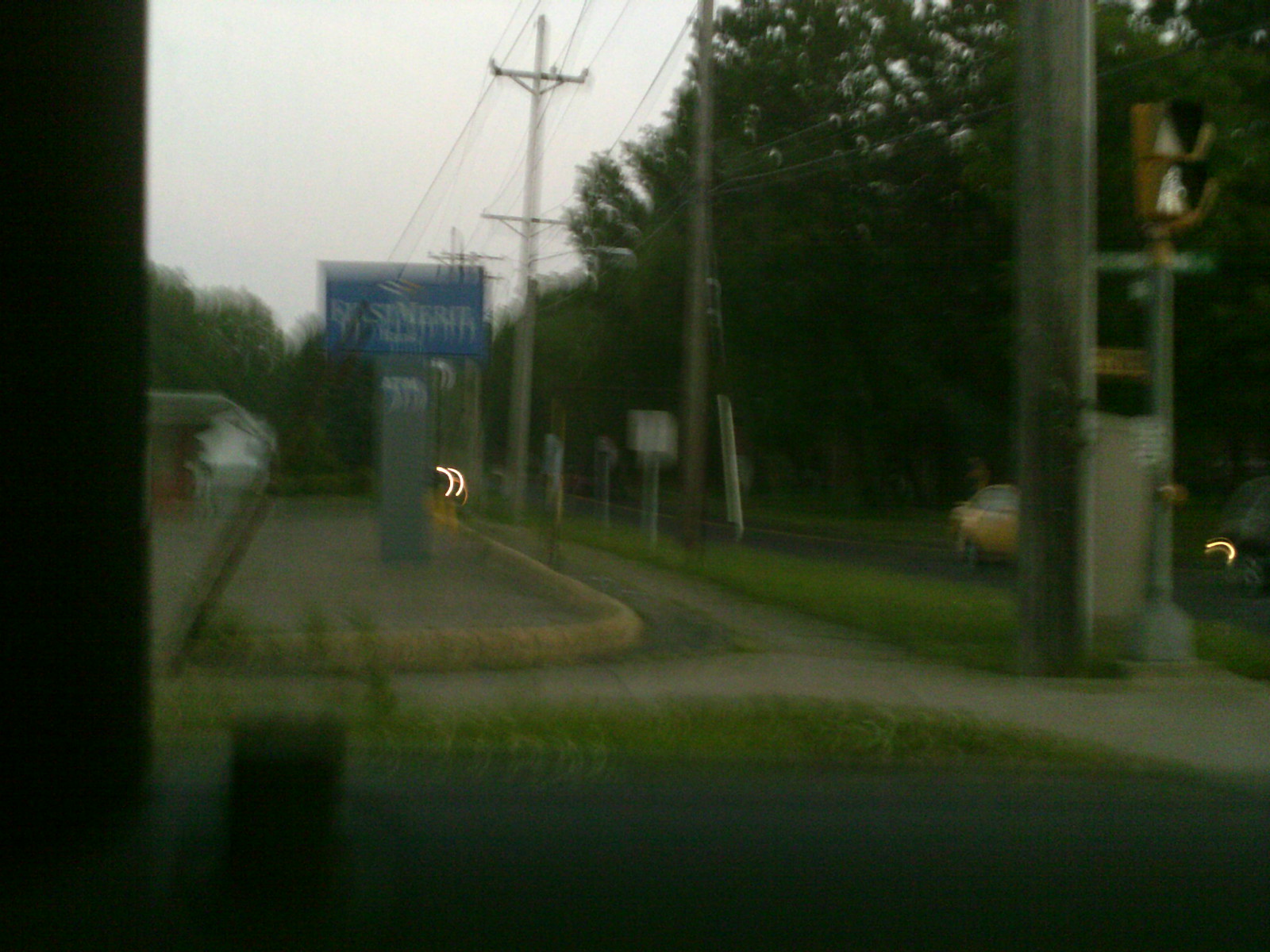A dimly lit, blurry outdoor photograph captures a sidewalk and street scene on an overcast day. The perspective is from a grassy area, looking towards a sidewalk and a roadway that stretches into the distance. Numerous telephone poles and connecting wires are prominently visible against a gray sky. On the right side of the scene, mature trees line the road, creating a natural border that extends into the horizon. Straight ahead, a blue rectangular bank sign on a square post with the white letters "ATM" is partially visible but indistinct due to the blur. A building partially emerges from the left side of the frame, adding to the urban elements of the setting.